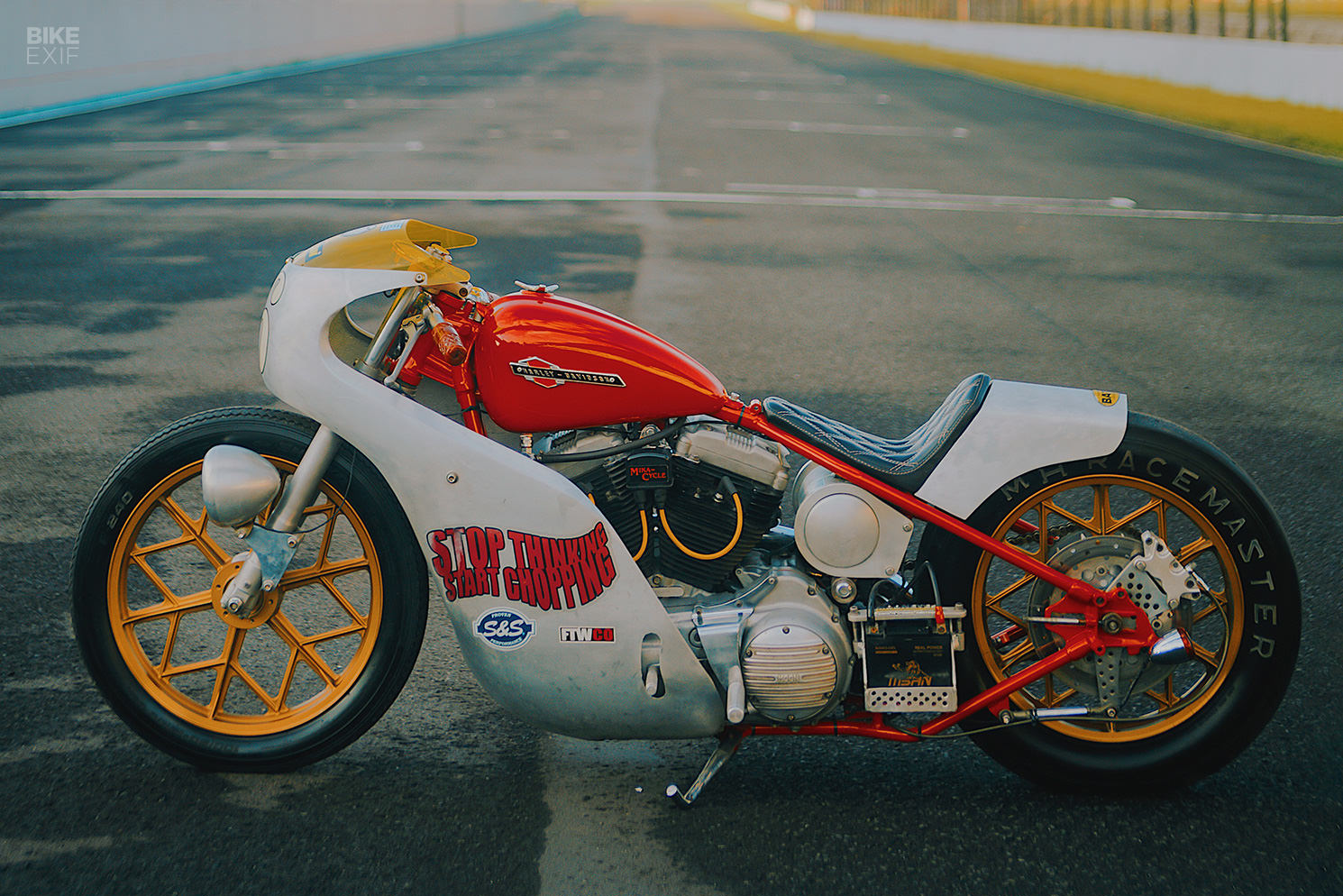The image features a detailed and vibrant racing motorcycle positioned horizontally on a track that stretches into the background. The track's upper right corner reveals a yellow border adorning a white wall that recedes into the distance. Prominently displayed on the bike's white side fender is the bold red slogan, "Stop Thinking, Start Chopping," further accompanied by a blue background with the letters "S&S" and "FTW Company." The motorcycle showcases a striking color palette: the gas tank is an eye-catching red, coupled with mustard yellow spokes on both the front and rear wheels. Red extension bars rise towards the gas tank and extend under the pedals, while the seat is a cool blue. Visible elements also include the motorcycle's battery on the left side. Completing the bike's aesthetic are yellow handlebars and a display windshield. The scene is brightly lit, indicating it's shot outdoors during the day, capturing the motorcycle set up centrally in an inviting, clear image, likely intended for advertisement purposes. The photo exudes clarity, perfect for showcasing the vehicle's intricate details to potential buyers.